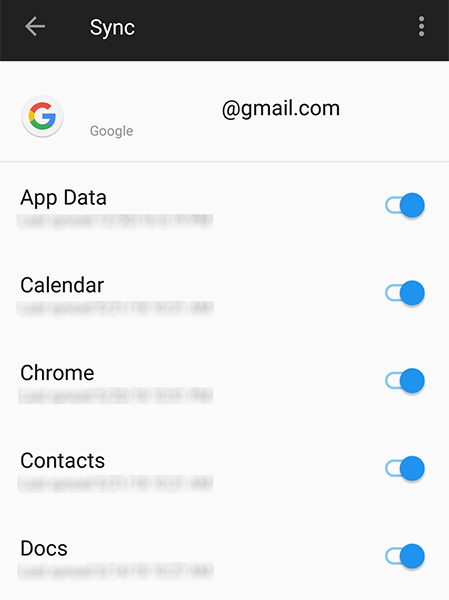Here is a cleaned-up and descriptive caption for the image:

---

This image displays a screenshot of the sync settings on a Gmail account. At the top, a black header features the word "Sync" in white text and a gray back arrow to the left. To the right, three vertical dots for additional options are visible. Immediately below this header, "Google" is written in gray letters accompanied by the colorful Google "G" logo in red, yellow, green, and blue, followed by the account's email address ending in "@gmail.com."

The screenshot lists various sync options, each accompanied by blocked-out data fields for privacy, with blue toggle buttons indicating that syncing is enabled. These options include:
1. **App Data** - Syncing is turned on.
2. **Calendar** - Syncing is turned on.
3. **Chrome** - Syncing is turned on.
4. **Contacts** - Syncing is turned on.
5. **Docs** - Syncing is turned on.